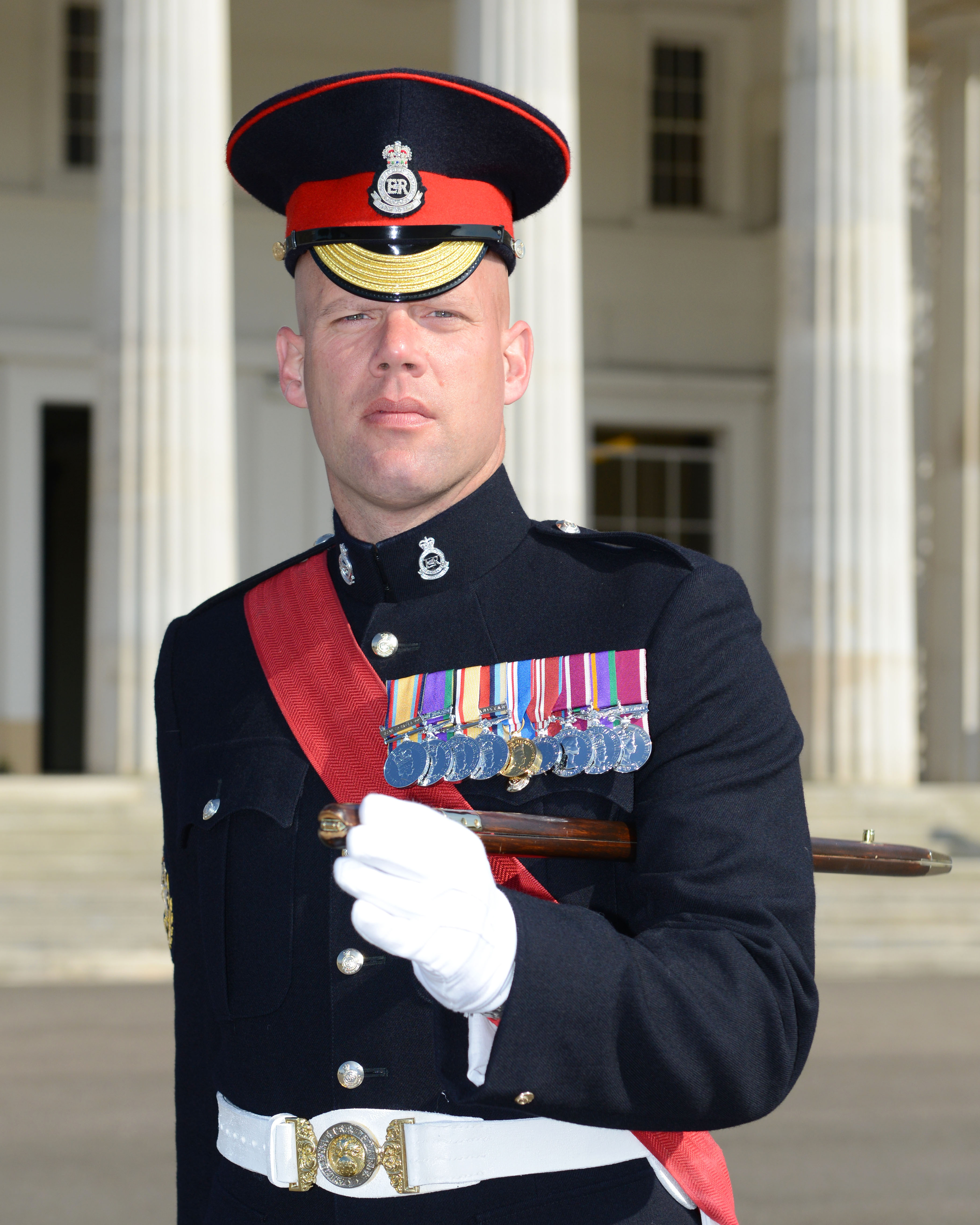The image captures a solemn soldier standing in front of a grand white building with large pillars, likely indicating an important location. The man is dressed in a meticulously detailed dark blue or black military uniform adorned with numerous brightly colored medals on the left side of his chest, and his rank and distinctions are prominently displayed. His uniform is distinguished by a red sash crossing from his right shoulder to his right hip and a white belt fastened with an ornate gold and silver buckle. He is wearing a high military hat with red stripes and a gold bill that features the Elizabeth Regina logo, suggesting his affiliation with the Royal British Army. His left hand, clad in a white glove, holds a wooden gun handle, and his arm is bent at his waist. The soldier stands with a dignified presence, looking directly into the camera, highlighting his decorated status and solemn demeanor. The overall scene reflects both the soldier's stature and the historical importance of the military setting.